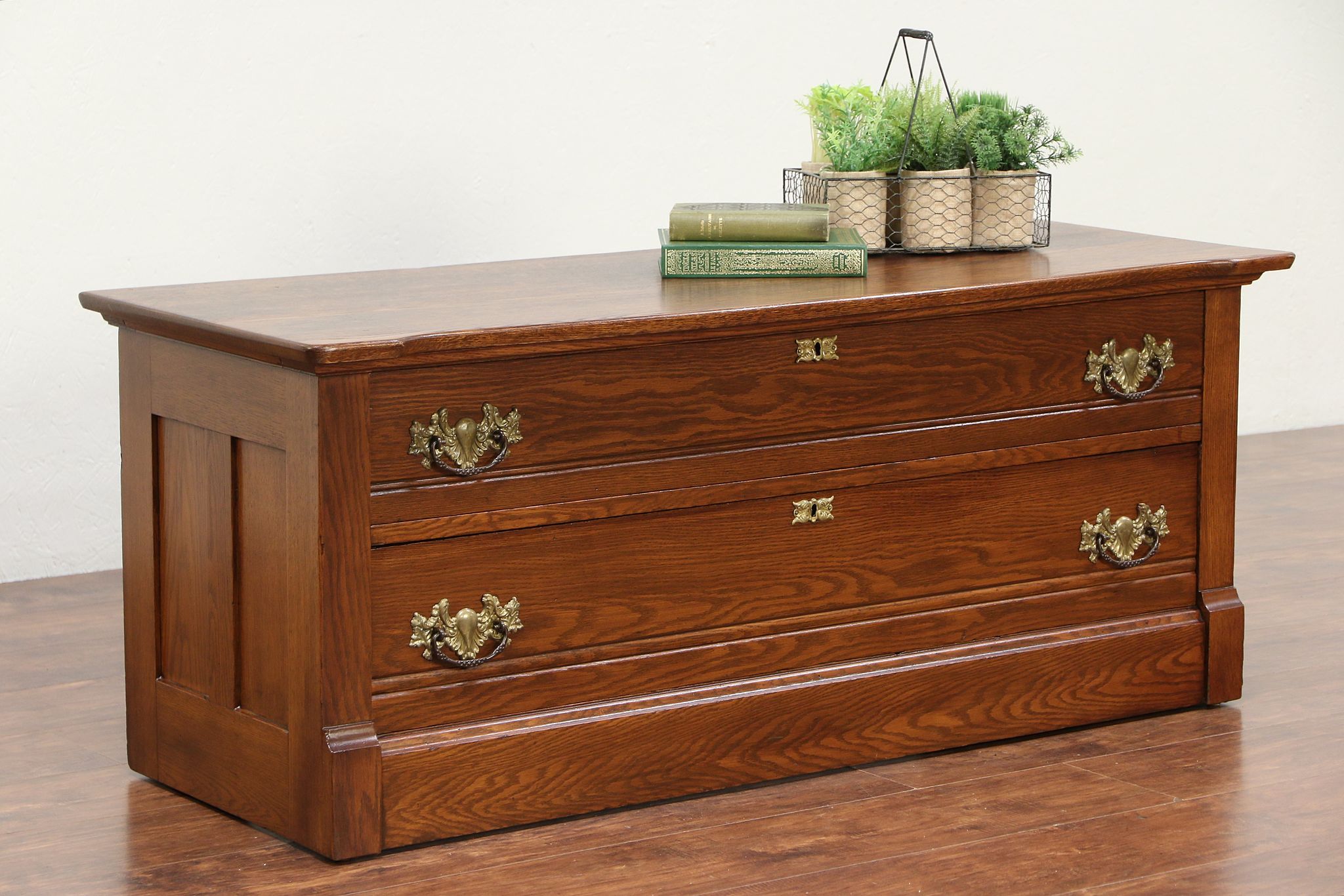The photo depicts a medium brown wood bureau standing on hardwood floors against a white wall. Despite its modest height of around 28 inches, its considerable width of approximately 5 feet makes it quite expansive. The bureau features two long drawers, each adorned with a brass keyhole in the center and two ornate brass handles on either side. The wood grain varies, showcasing v-shaped and tiger stripe patterns. On top of the bureau sit two vintage-looking green books, reminiscent of those found in a Victorian library, alongside a small wire basket filled with potted ferns and succulents. The furniture's polished finish and golden handles add an elegant touch to the room's decor.